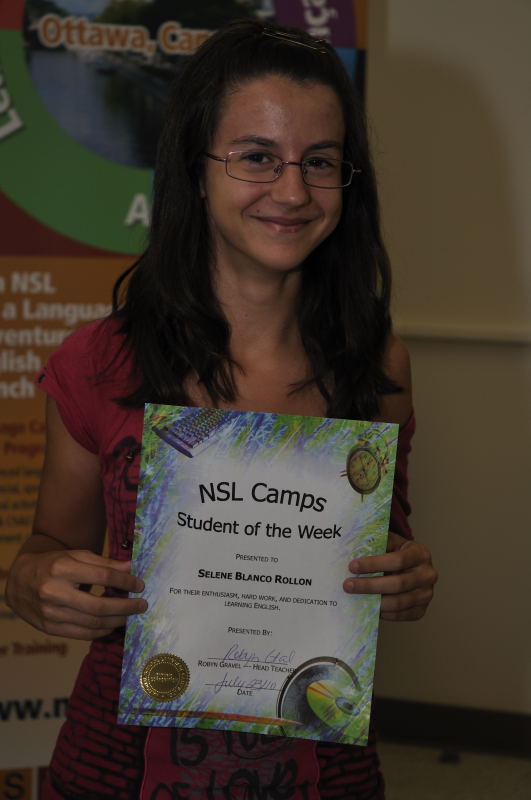This photograph captures a young girl, approximately 13 years old, with long dark hair and eyeglasses, smiling and posing for the camera. She is wearing a sleeveless red dress and proudly holding up a certificate that reads, "NSL Camps Student of the Week, presented to Selene Blanco Rowland." The certificate features a gold seal on the left side and signatures at the bottom, along with illustrated elements, including a flying saucer on the lower right, a clock in the upper right, and a keyboard in the upper left. The background features a dingy yellow wall adorned with various posters and signs, including one partially obscured poster with the text "Ottawa" visible.